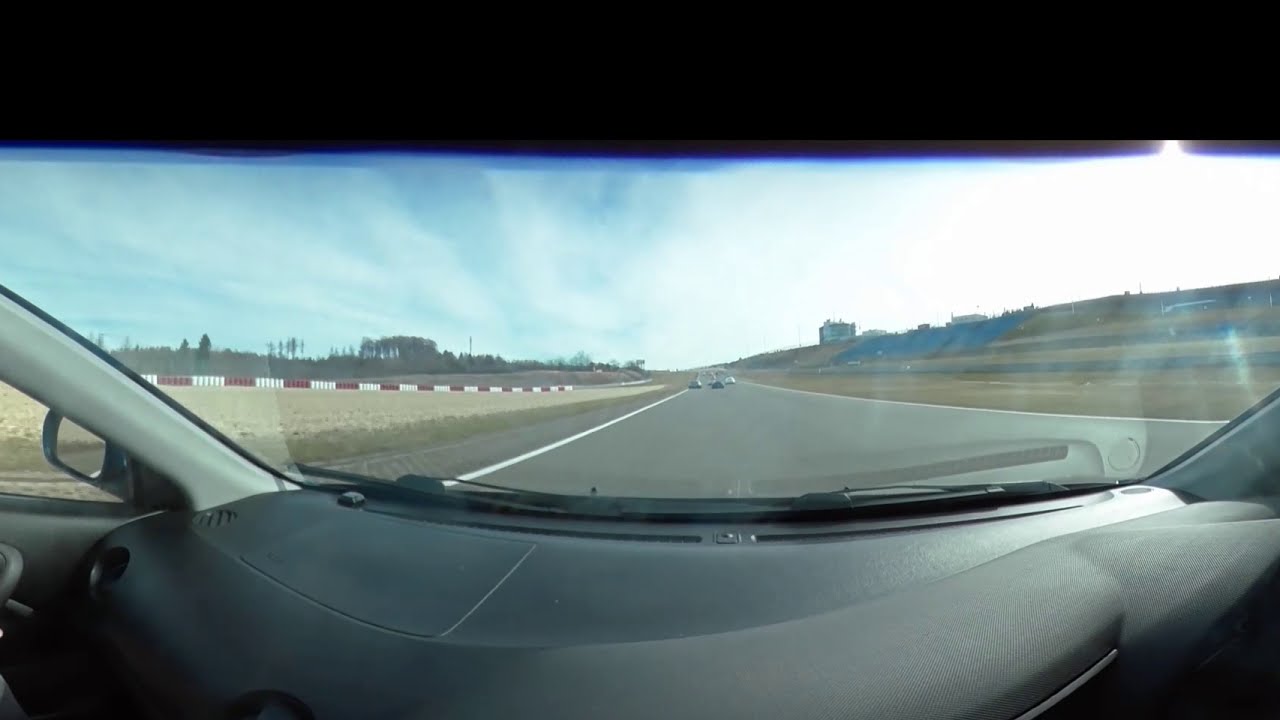The photograph, taken from within a car through the windshield, captures a moment on a professional driving track under a blue but cloud-dragged sky. The interior view reveals a black dashboard and a sun reflection on the windshield. The track, wide enough for about three cars abreast and lacking lane markings, stretches ahead with a few cars visible in the distance. On the right side of the image, blue-painted spectator stands built into a hillside are seen, while the left side features safety barriers and medians. The track is bordered by dull green and brown grass, suggesting a time outside of summer. The scene is further framed by a sparse treeline.